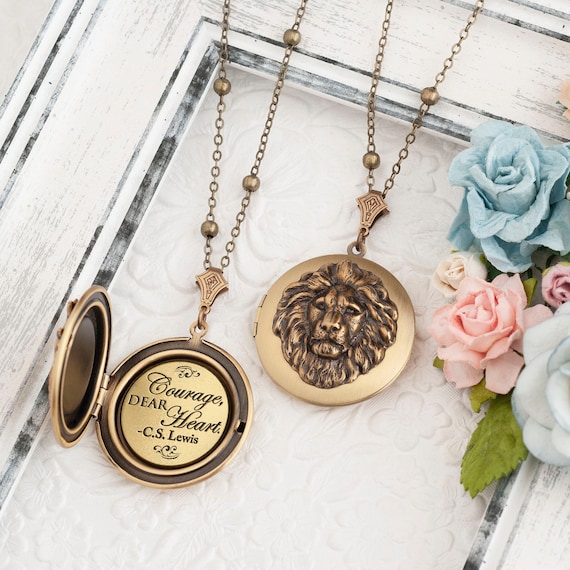This photograph showcases two gold lockets, each hanging from a delicate gold chain, draped over what appears to be a picture frame with black trim. In the upper right-hand corner of the frame, there is a beautifully arranged bouquet of roses, featuring a dominant blue rose, a pink rose underneath, a white rose to the right, and interspersed with a few smaller pink rose buds and some green foliage. The left locket is open, revealing an inscription inside that reads, "Courage, Dear Heart, C.S. Lewis." The right locket remains closed, displaying an intricately engraved lion's head with a voluminous mane, giving the piece a majestic and ornate appearance. Both lockets possess a slightly tarnished patina, adding to their vintage charm.